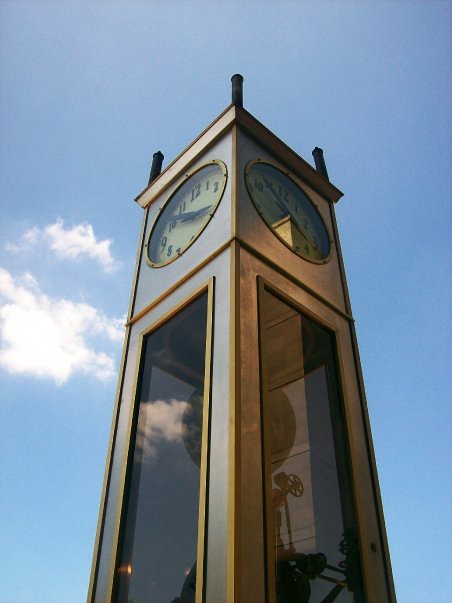This photograph captures a striking, tall clock tower set against a bright blue sky punctuated by a few small, wispy white clouds on the left. The tower, constructed from smooth grey stone, is imposing and rectangular, accented with golden metal edges that impart a sense of elegance. At the top of the tower, on all visible sides, are large white clock faces encased in glass, each adorned with black numerals and hands, clearly indicating the time. Below these clock faces, clear glass pane windows are set into the stone, allowing a peek into the clock's intricate internal mechanics. The reflection of the sky and clouds can be seen on these glass panes, enhancing the tower's majestic appearance. Each surface of the tower features these glass windows, bordered by thin brass, revealing the meticulous design elements that harmonize both functionality and aesthetics.